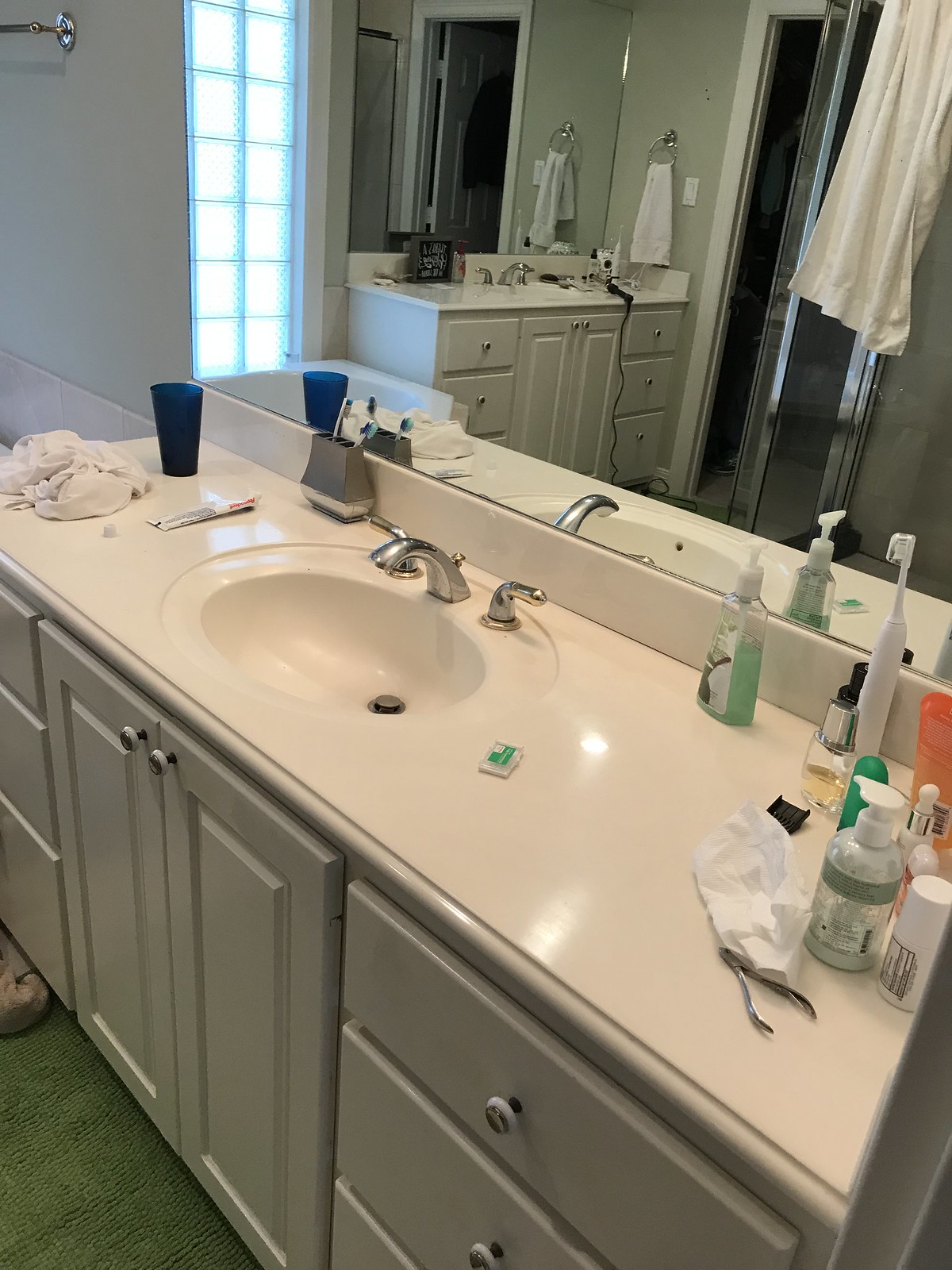The close-up photo showcases a pristine bathroom sink with a completely white finish, extending through the bowl and the accompanying cabinetry. The cabinet includes two central doors, flanked by three partially-visible drawers on each side. Above the sink, a mirror reflects the rest of the bathroom, adding depth to the scene.

To the left of the sink basin, a blue cup sits near the mirror, accompanied by a balled-up white cloth and a tube of toothpaste. Nearer to the sleek faucet and handles, a gray container houses several toothbrushes. The right side of the sink features a plastic hand soap dispenser filled with green soap, positioned beside a white electric toothbrush. In front of these, numerous bottles clutter the countertop, their specific contents difficult to identify. Among them lie a pair of tweezers and a small paper wrapper.

Additionally, a glimpse of the textured grayish-green floor is visible in the bottom left corner, completing the setting of this meticulously detailed bathroom scene.